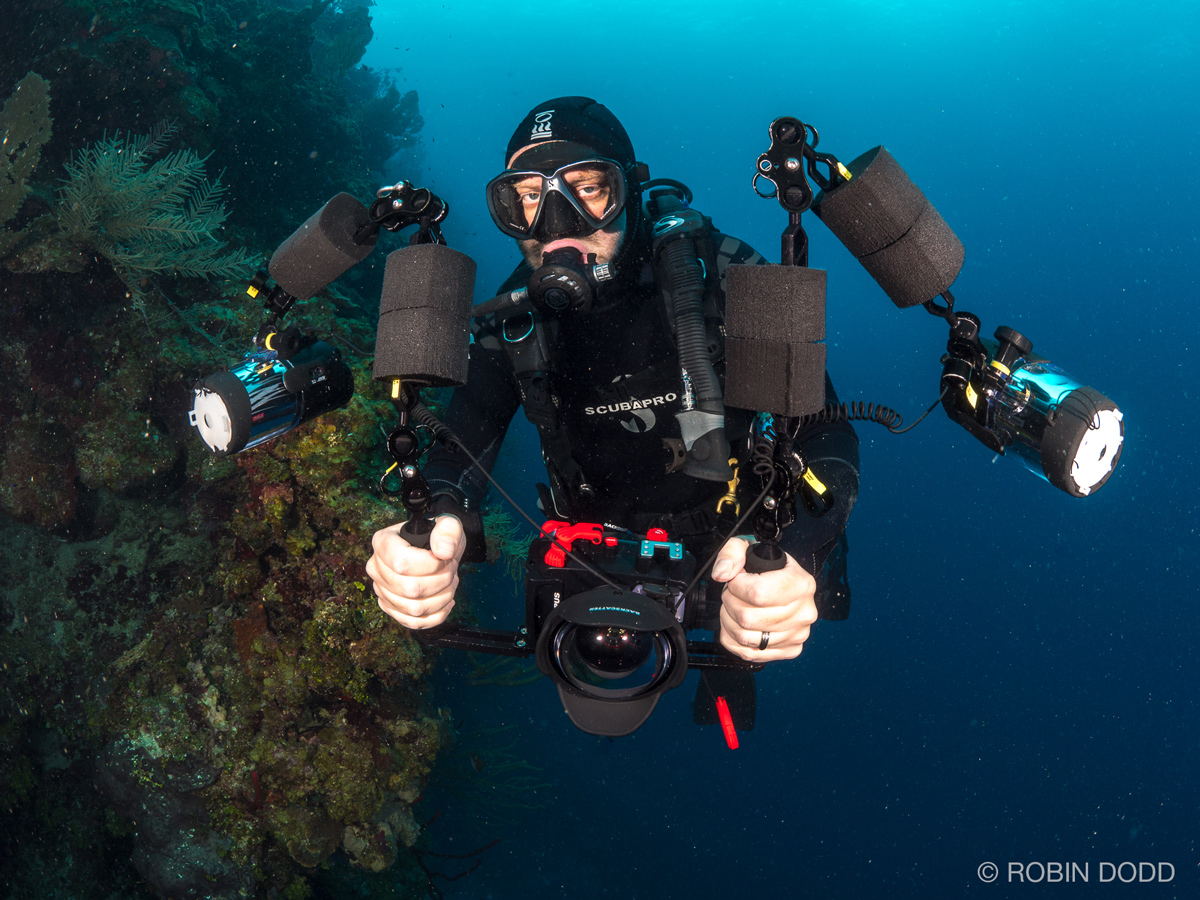This captivating underwater photograph, credited to Robin Dodd, features a scuba diver immersed in the deep, dark depths of the ocean, illuminated by his advanced diving equipment. The diver, clad in a black scuba suit, mask, and tank, wields an intricate setup consisting of a large camera flanked by two sizable, weighted lights. These lights are steered with handles, allowing for a wide range of directional illumination, highlighting the vibrant coral reef drop-off teeming with vegetation, coral, and algae. The vivid red parts on the camera and the yellow reflective components on the lights add a touch of color to the otherwise monochromatic gear. The diver, ring visible on his bare hand, appears focused, directing his gaze towards another individual capturing this breathtaking scene. Above, the faint light from the ocean's surface contrasts with the eerie darkness below, emphasizing the depth of this stunning underwater realm.